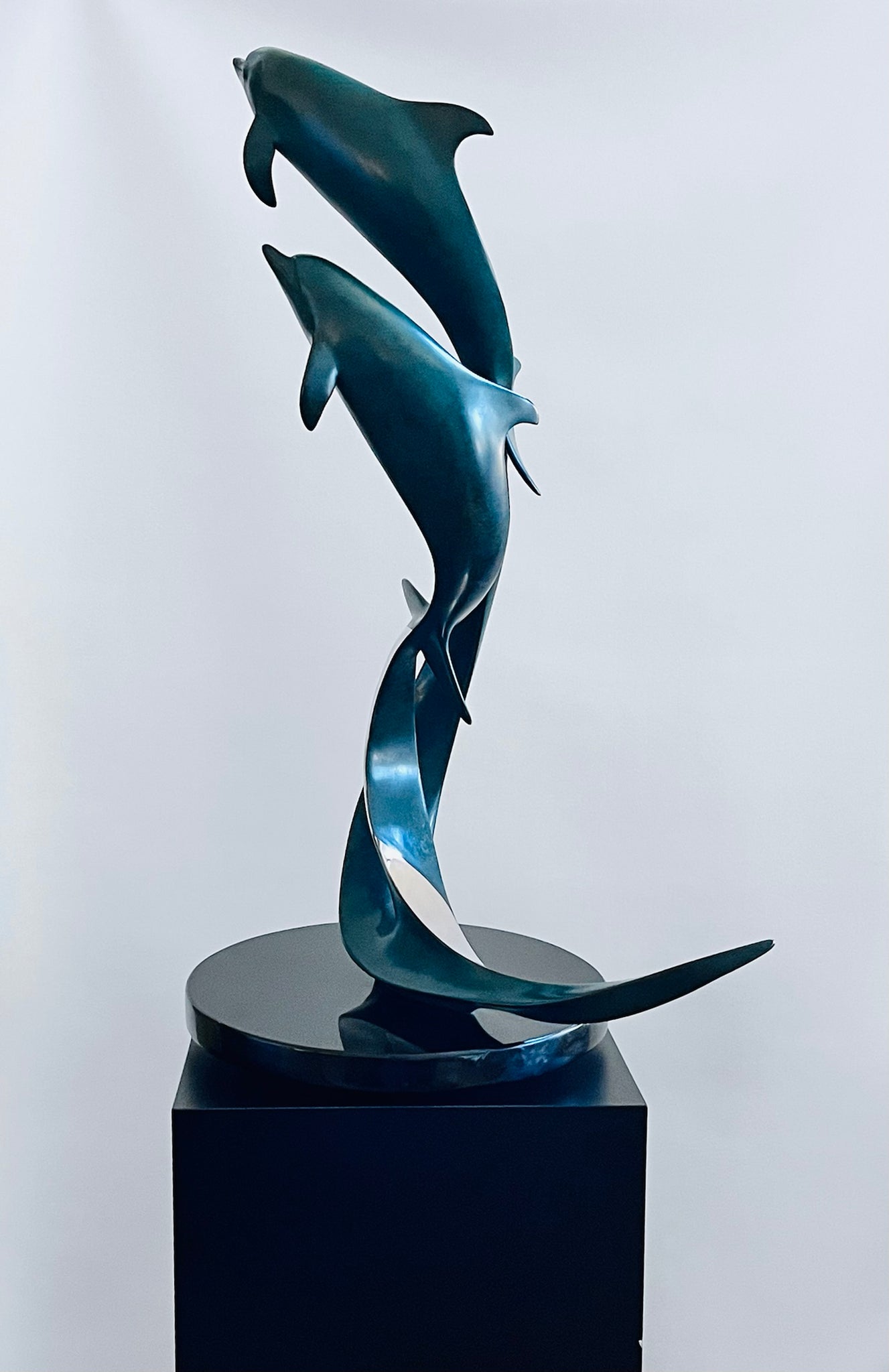This detailed image depicts an indoor setting, potentially a museum. At its center is a polished black metal base, comprising a rectangular block with a circular top. Rising from this base is a sculpture featuring two blue dolphins, elegantly designed to look like they are swimming toward the ocean's surface. These dolphins are turned away from the camera, showcasing their top and side fins. They are connected to the base via a sweeping element that transitions in shades of blue and gray, resembling water. The sculpture stands out against a light gray background and contains no text. The overall composition is centered within the image, highlighting the intricate details and movement of the marine-inspired artwork.